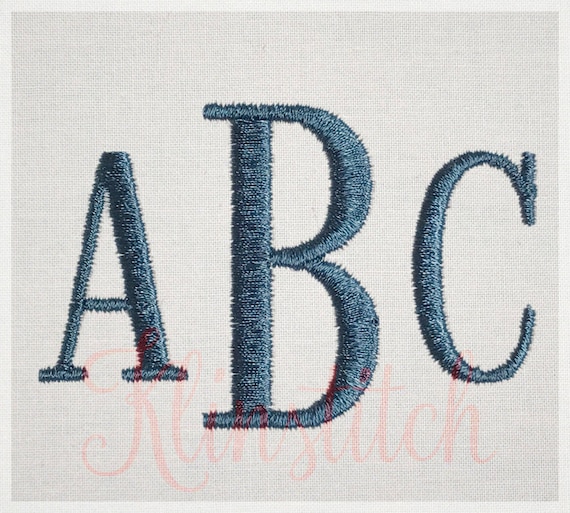This square image features a beige or light gray fabric background bordered by a thin pale strip. Centered on this textured backdrop are the embroidered capital letters A, B, and C, created with a rich, dark blue thread. The letter B is the largest, making it the focal point, while the A and C, both smaller, are positioned to its left and right, respectively. Beneath these letters, a faint, cursive watermark in a very light, almost pinkish hue reads "K-L-I-N-S-T-I-T-C-H," indicating the likely name of the creator or brand. The detailed stitching and the contrast between the blue letters and the soft pink watermark add a sophisticated touch to this textile piece.